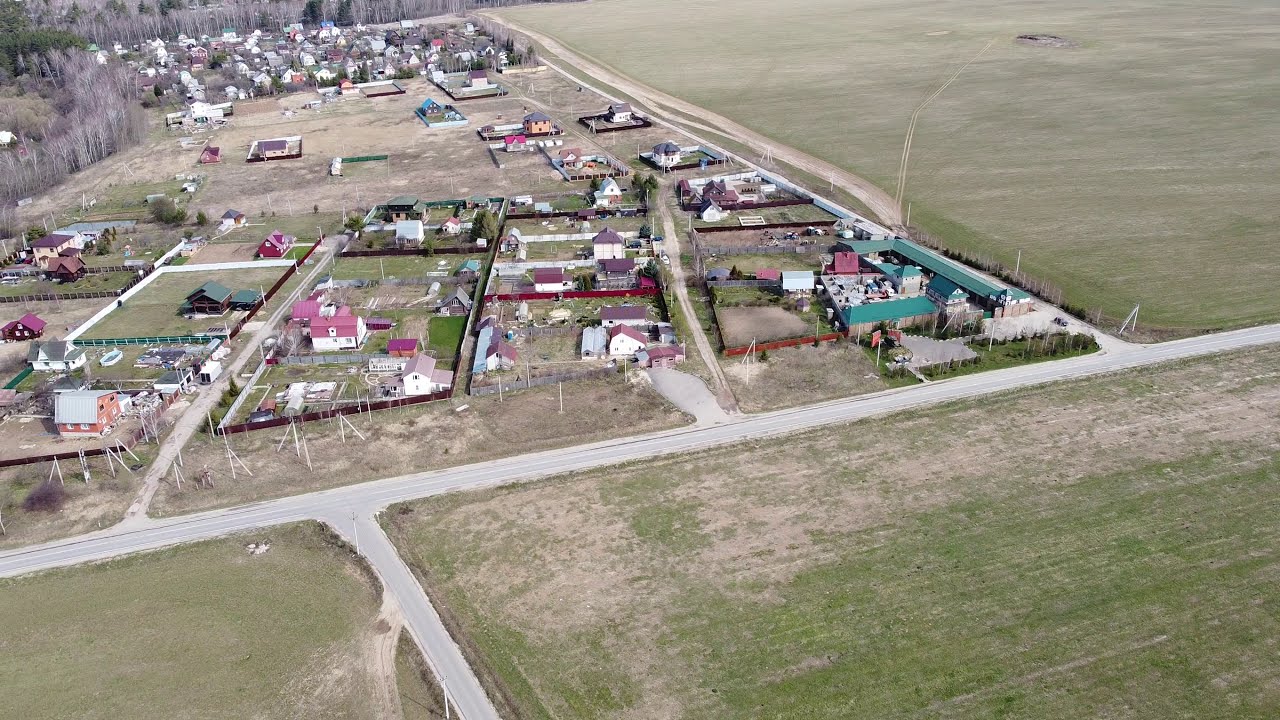An aerial photograph captures a small European town, characterized by a network of roads and residential areas. At the core, a two-lane paved road traverses from the middle right to the bottom left, branching off in two directions — one leading to a smaller, one-lane dirt path on the right, and the other veering toward the top left. This dirt path showcases a cluster of houses, each with fenced plots of varying sizes and colors, surrounded by ample yards. To the right of the main road lies a vast, tan-colored open field, possibly used for agriculture. The town is enveloped by dense clusters of trees in the distance, further enhancing its pastoral charm.